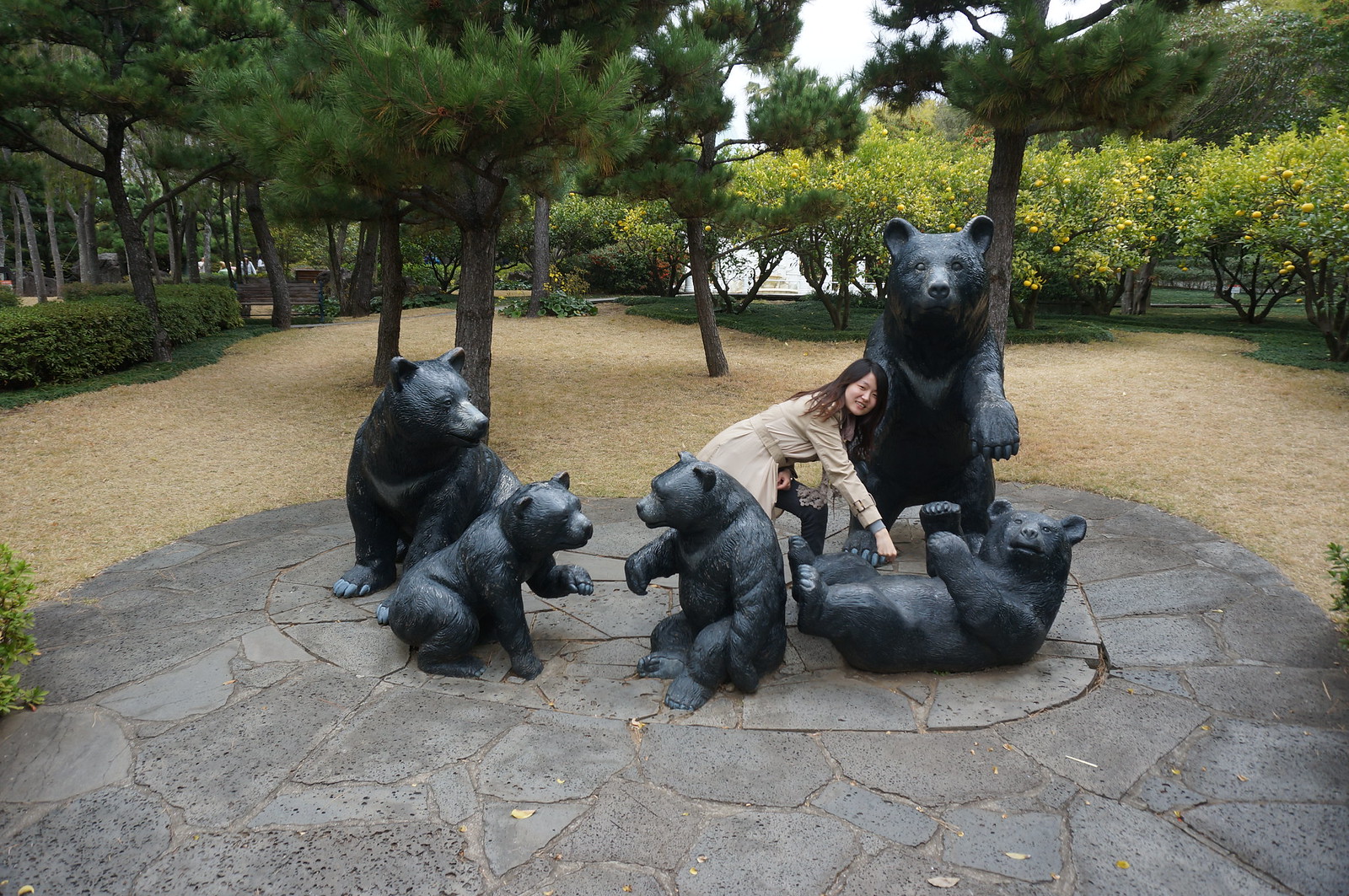In this bright, overcast photograph set in a tranquil park, a woman with long brown hair, dressed in a tan coat, is joyfully interacting with a charming arrangement of bear statues. The scene features a family of bears—painted in deep black with gray accents on their snouts—positioned on a central stone path amidst a clearing surrounded by evergreen trees and lush bushes. In particular, the woman is playfully posing with one bear cub lying on its back with its limbs in the air, as if inviting a belly rub. The statues include a standing father bear towering next to the woman, a seated mother bear off to the left, and two cubs engaging with each other near the center. The ground underneath the statues consists of dark and light gray stones interspersed with soil, and around this arrangement, the ground is strewn with hay or pine needles, with wood chips forming a light tan area behind the playful scene. This delightful park setting is further enriched by yellow blooms on surrounding hedges, adding vibrant touches to the serene landscape.